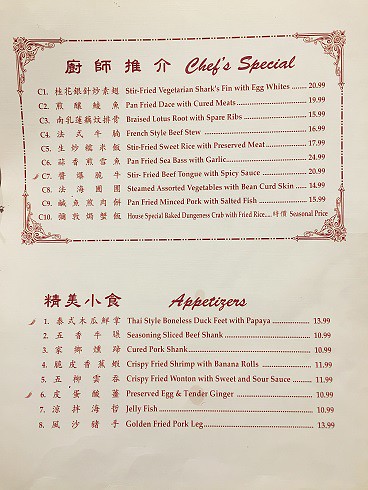This image captures a detailed view of a restaurant menu set against a beige sheet of paper. The menu is organized with a red-bordered box on the right side, featuring ornate decorations at its corners. Within this box, the heading reads "Chef Special," followed by a list of dishes numbered from C1 to C10. Each dish is described with its name written first in Chinese characters and then translated into English, alongside their respective prices. Notably, the entry for C7 includes a small chili icon, indicating a spicy dish.

Below the "Chef Special" section, the menu lists "Appetizers" without a boxed border but maintaining a similar format. The appetizers section features numbers from 1 to 8, also presented with Chinese names on the right and English translations on the left. Prices for these dishes are clearly marked. Dish number 1 and dish number 6 both have a small chili icon next to them, signifying that these items are spicy offerings. The entire menu layout combines clarity and elegance, making it easy for diners to select their desired dishes.